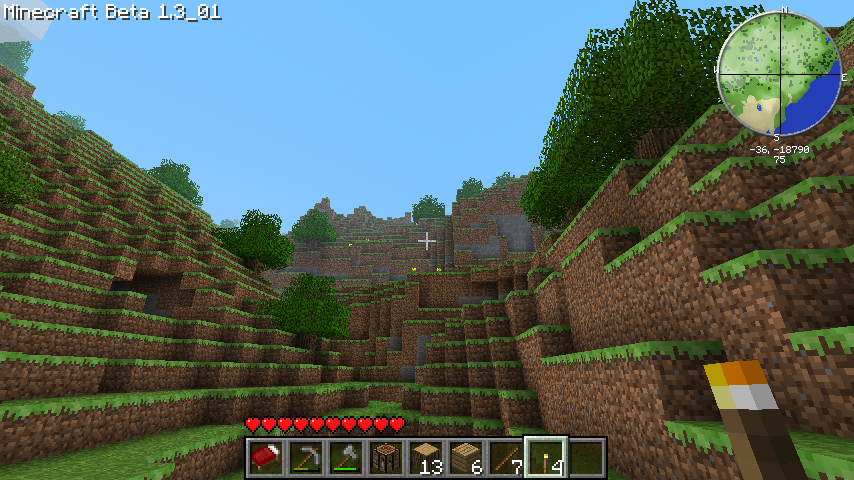In this captivating Minecraft scene, we find ourselves nestled in the center of a grassy, dirt-filled hole. Numerous dirt blocks with lush green grass on their tops surround the area, creating a naturally enclosed environment. On the left side, a significant portion of dirt blocks has been removed, revealing a large gap in the hillside. To the right, a sturdy rock wall rises, adding a rugged texture to the scene. 

Amidst this earthy setting, an adventurer's gear is scattered strategically. A cozy bed sits prominently, alongside a handy crafting table. The player's inventory reveals 13 logs, 6 wooden planks, and 7 branches, probably gathered for future crafting sessions. Essential tools like a pickaxe and an axe lie ready for use, while 4 torches illuminate the area, with one currently held, casting a warm glow. 

Above, a lone tree stands in the top right corner, its leafy canopies reaching out against the sky. In the distance, vibrant yellow flowers dot the landscape, adding a splash of color to the verdant surroundings. The scene is a harmonious blend of nature’s beauty and a prepared explorer’s domain, captured in a moment of tranquil readiness.